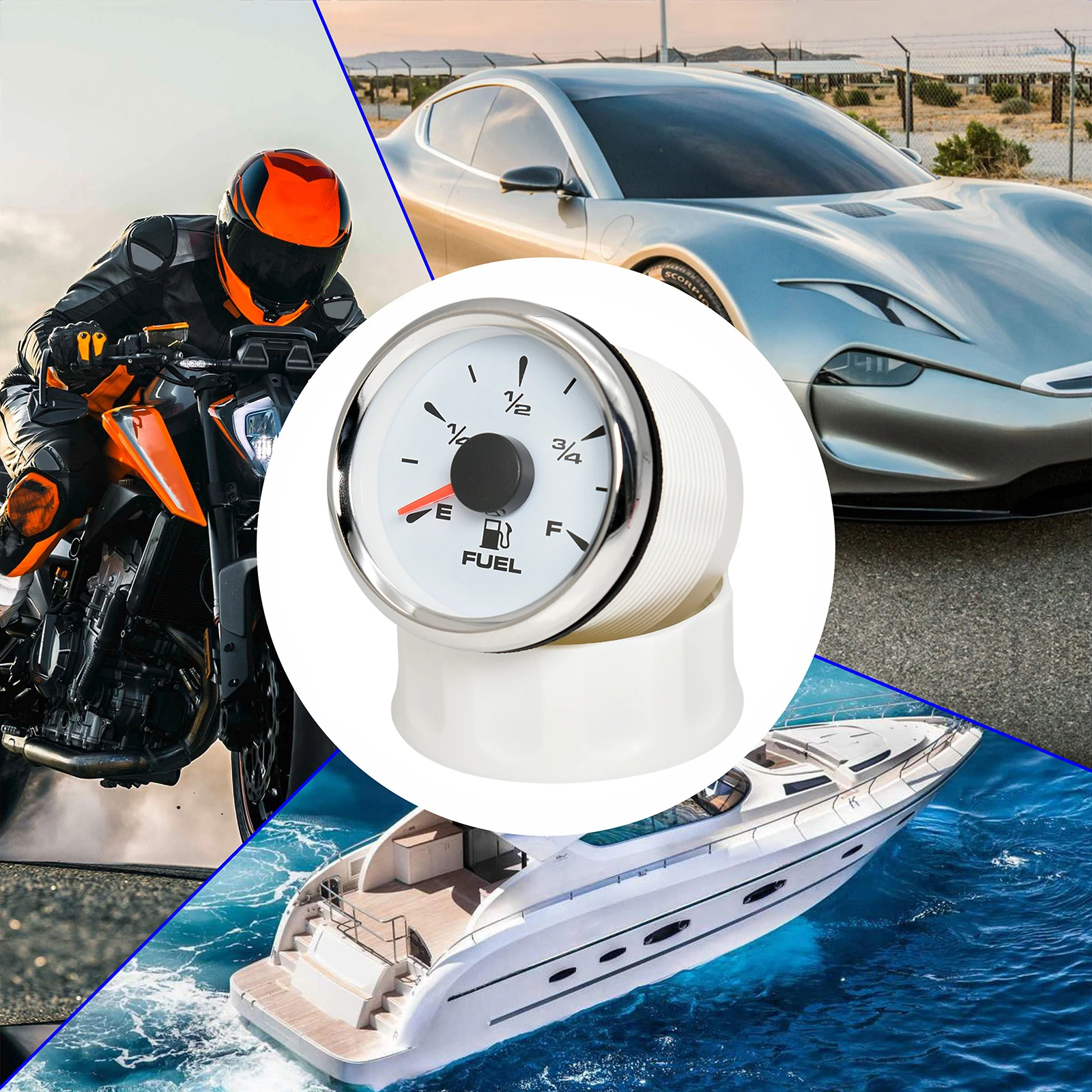This collage artfully combines four distinct images into a visually cohesive composition, highlighting elements of luxury and adventure. In the top left quadrant, a solo biker rides a sleek black and orange motorcycle. The biker sports a matching orange and black helmet, with black leather gear accented by orange pads, all set against a white backdrop with a hint of a light blue to gray sky. Adjacent to this, in the top right, a pristine silver sports car is showcased, parked on asphalt against a serene desert landscape that features hills, sparse greenery, and a distant fence.

The bottom portion of the collage features a vibrant, blue ocean occupied by a luxurious white yacht, adorned with black stripes and large windows, suggesting a warm, tropical locale. At the center of the collage, overlaying parts of these three images, sits a circular fuel gauge. This silver gauge with a white face and an orange needle strikingly indicates empty, possibly alluding to the energy demands of these portrayed vehicles. The thoughtful merging of these images creates a dynamic visual narrative of high-end travel and adventure interlinked by the essential need for fuel.